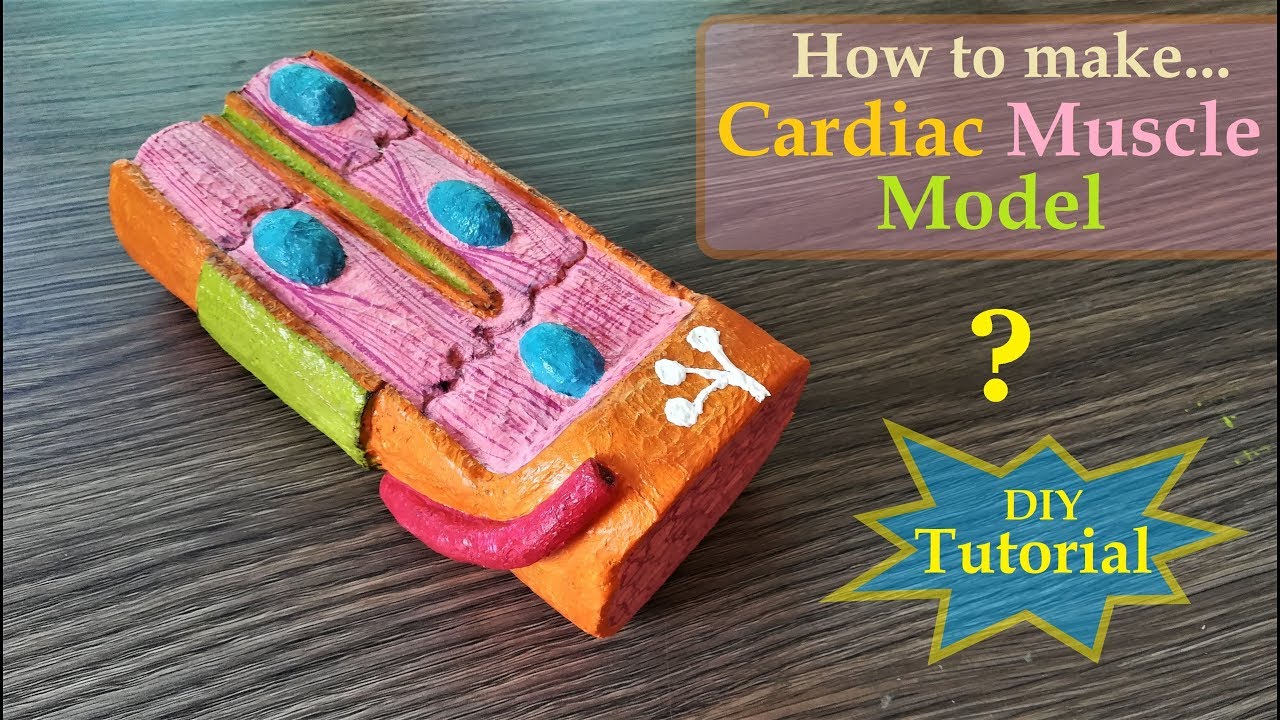In this horizontally-oriented photograph, a detailed illustration of a "How to Make Cardiac Muscle Model" DIY tutorial is depicted on a wooden surface. The title, "How to Make... Cardiac Muscle Model," is prominently displayed in light yellow, with "cardiac muscle" written in a gradient of yellow and light pink, and "model" in lime green. This text is surrounded by a partially transparent pink background with an orange border.

The central object is a meticulously constructed model of a cardiac muscle cell, made from various colorful materials. The main structure is an orange rounded rectangle with intricate inner details, including long pink lines likely representing the muscle fibers, and blue ovals symbolizing cell nuclei. A central lime green line extends two-thirds of the way down the model, and a matching lime green section is present on the side of the orange rectangle. 

Attached to the model is a bright pink hose, simulating a blood vessel, which curves from the bottom to the top of the structure. Additional features include an orange-highlighted three-pronged item and orange elements that add further detail to the representation. A prominent blue star, outlined in green, features the text "DIY Tutorial" near the top right, enhancing the instructional nature of the image. A bold yellow question mark is also noticeable in the lower right corner, accentuating the educational intent of the tutorial.